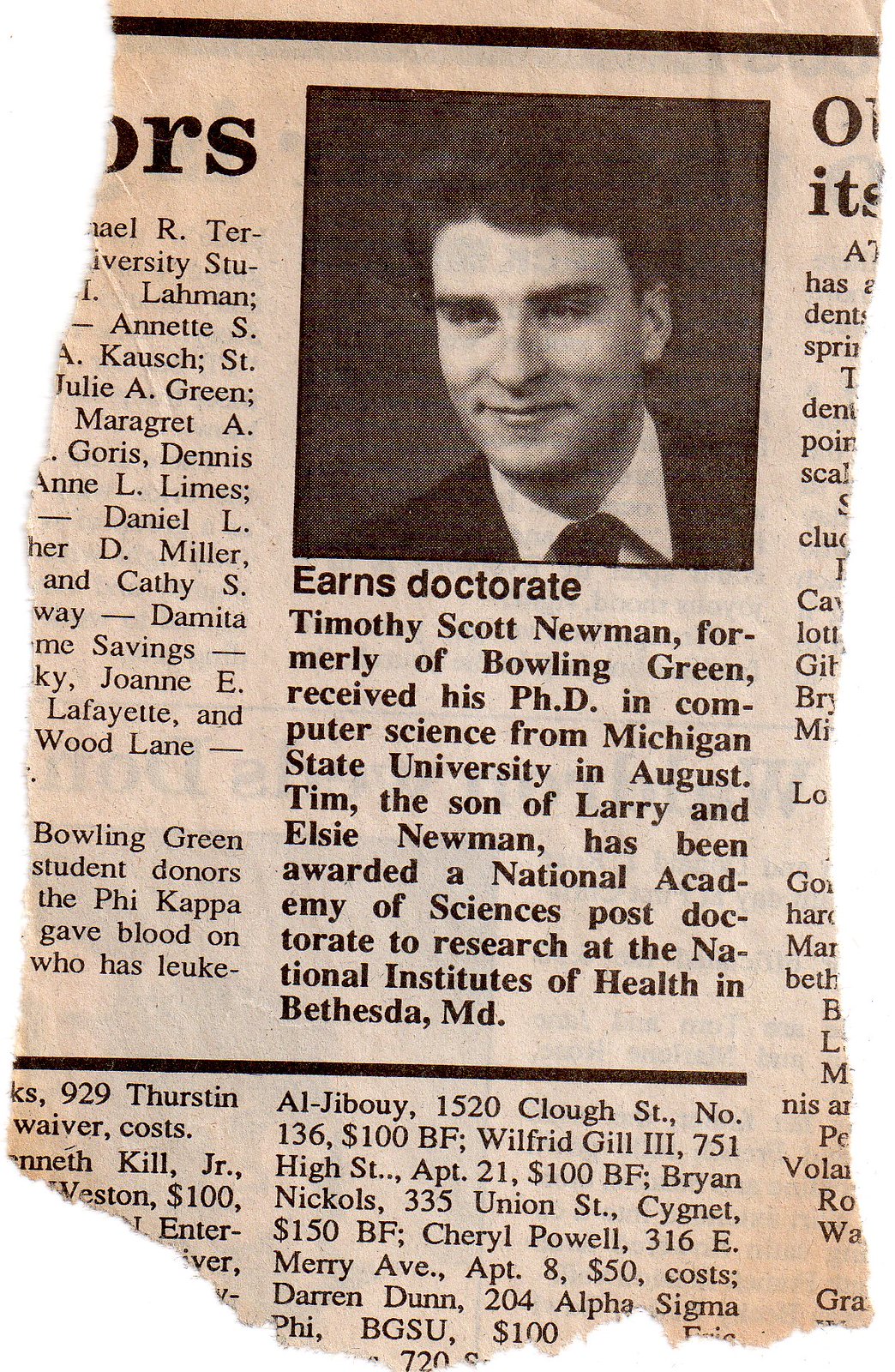The image depicts a jagged-edged newspaper clipping, seemingly torn with care from a larger page, with partial remnants of other articles bordering the edges. Dominating the forefront is a black-and-white photograph of a young man, Timothy Scott Newman, dressed in a suit and tie and smiling directly at the camera. The headline beneath the photo proudly states, "Earns Doctorate." The accompanying text details Timothy Scott Newman's recent achievement, noting that he hails from Bowling Green and has been awarded a Ph.D. in Computer Science from Michigan State University in August. The announcement further highlights that Tim, the son of Larry and Elsie Newman, has been granted a National Academy of Sciences post-doctorate fellowship to conduct research at the National Institutes of Health in Bethesda, MD. The clipping appears to hold sentimental value, serving as a cherished memento of Timothy's significant academic milestone. For further information, a web address, www.fema.gov, is provided, although its relevance to the announcement is unclear.